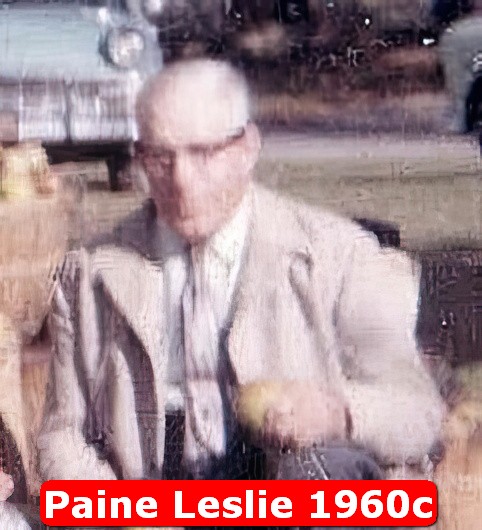This is a very blurry, out-of-focus photograph from 1960, identified by the text "Payne Leslie, 1960C" in a red banner with white lettering at the bottom. The central figure is an elderly white man, likely named Payne Leslie, given his appearance in the photo. He has white hair and wears black glasses, a light-colored (possibly beige or gray) coat, a white shirt, and a silver or gray tie. He appears to be sitting outdoors, possibly in a motorized chair or wheelchair, holding a device in his hand. The background reveals a road with a few cars, including a light blue vehicle, suggesting the image was taken near a traffic area.